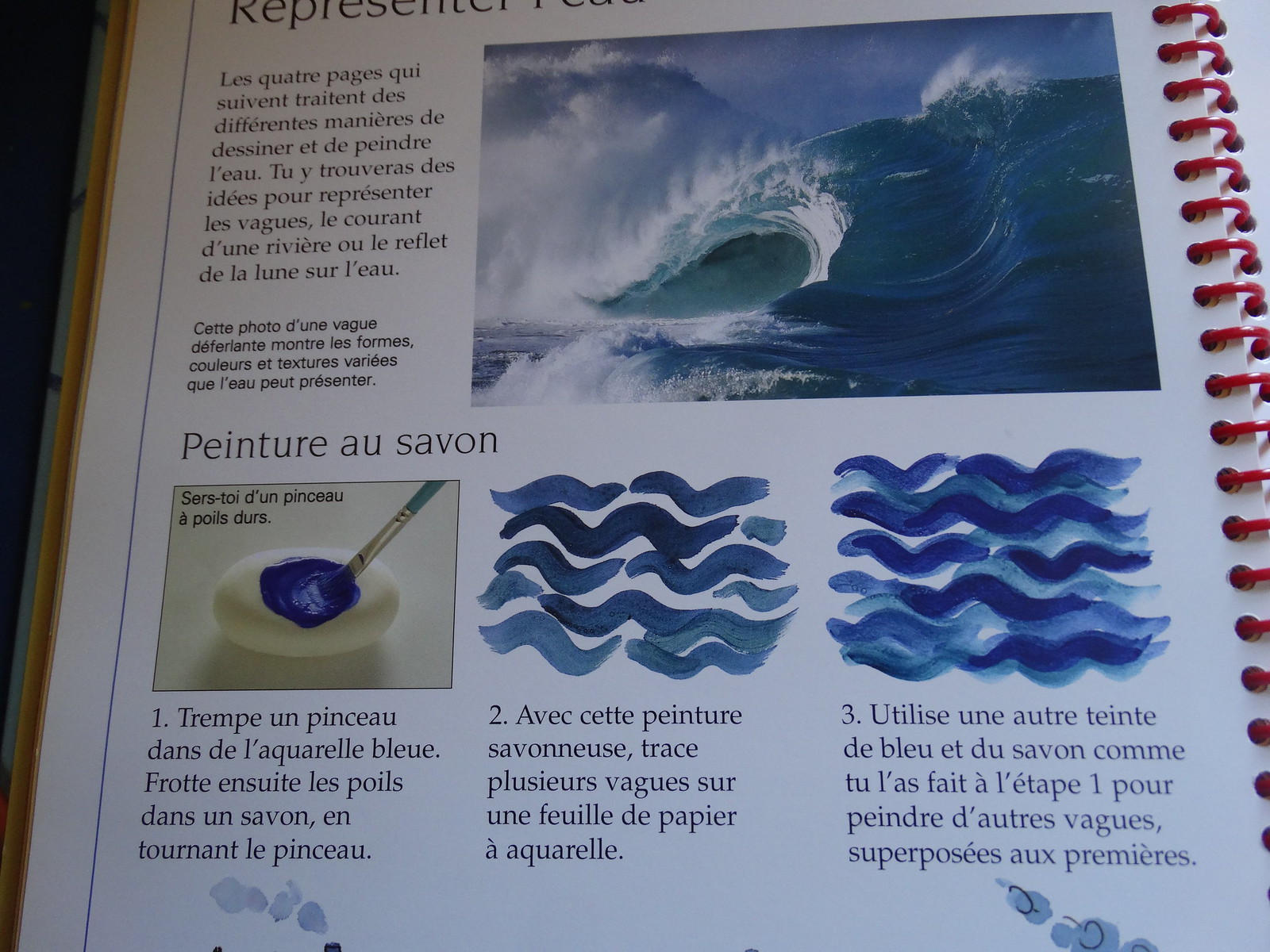This page from a spiral-bound book with red spirals down the right side appears to offer painting techniques, primarily focused on depicting waves. The top section features a dramatic photograph of large, crashing ocean waves. Adjacent to this photograph is a French dialogue box and a detailed paragraph. Below the text are three step-by-step illustrations: the first shows a paintbrush coloring a white circular object, likely a stone or egg, blue; the second highlights various shades of blue wavy lines; and the third continues with more intricate, squiggly lines of paint. All the instructional text is in French, suggesting this is an educational guide for painting water textures, with the real wave image provided as a reference.